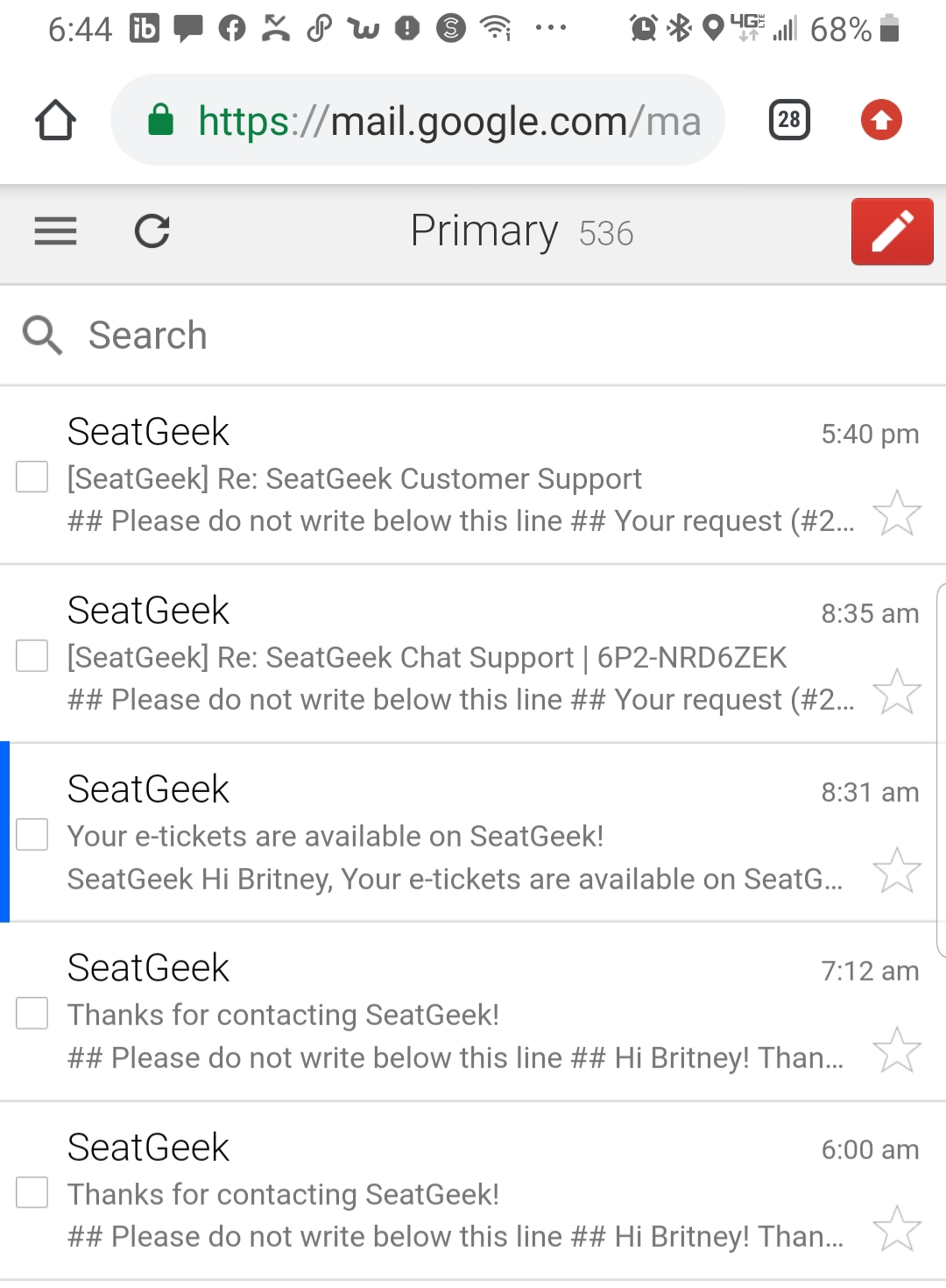In this image, a cell phone screen is displaying an email application. At the very top of the screen, a series of cell phone icons are visible from left to right: the time displayed at 6:44, a messaging icon, a Facebook icon, a voicemail icon, a Wi-Fi signal indicator, an alarm symbol, a Bluetooth icon, a location marker, and finally, the signal strength bar. On the top right corner of the screen, the battery percentage is shown at 68%.

Below the icon strip, there's a URL bar accompanied by an indicator showing 28 open tabs and a red circle featuring an upward-pointing white arrow, which likely indicates a file upload or sending action.

The main portion of the screen is dedicated to the email application. At the top of this section, the primary inbox is displayed, showing a count of 536 emails. On the left side of this bar is a refresh icon and a tab menu, while on the right, there is a prominent red button labeled "Compose."

Directly below this navigation bar is a search bar for finding specific emails. Underneath, the inbox shows five emails from the company SeatGeek. The first two emails state, "Please do not write below this line your request." The third email greets the user with, "Hi Brittany, your e-tickets are available on SeatGeek." The fourth email partially repeats the greeting: "Please do not write below this line. Hi Brittany, THAN," and the fifth email continues in a similar manner: "Please do not write below this line. Hi Brittany, same thing." 

The times of the emails are aligned on the right-hand side of the screen. A blue scroll bar is positioned approximately in the center of the screen on the left side, indicating the user's position within the inbox.